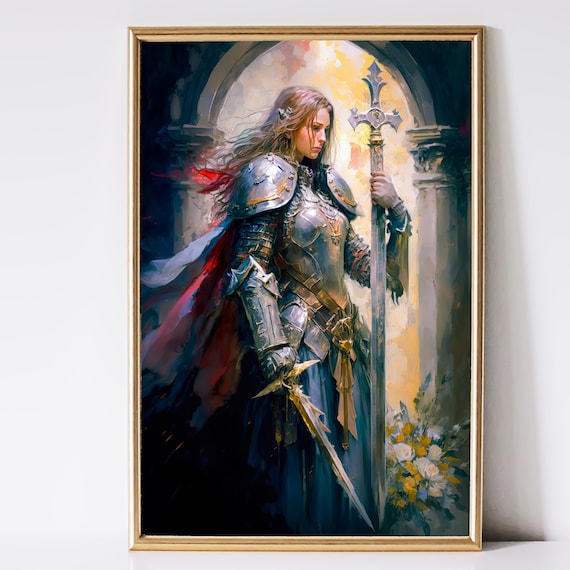The image features a framed painting leaning against a white floor and wall. The frame is a light gold color, not too thick, and encloses a detailed oil painting of a woman in a full suit of gray metal armor. She has long, flowing blonde hair, which appears to be blown back, and is adorned with a red and blue ribbon. Her armor covers her shoulders, bodice, and hips. In her right hand, she holds a small sword, while her left hand grasps a very large sheath extending almost her entire height. Her expression is one of sorrow, with pursed lips and sad eyes. In the background, there's an arched window or door letting in light, and white and yellow flowers are visible in the bottom right corner, adding a touch of softness to the somber scene.